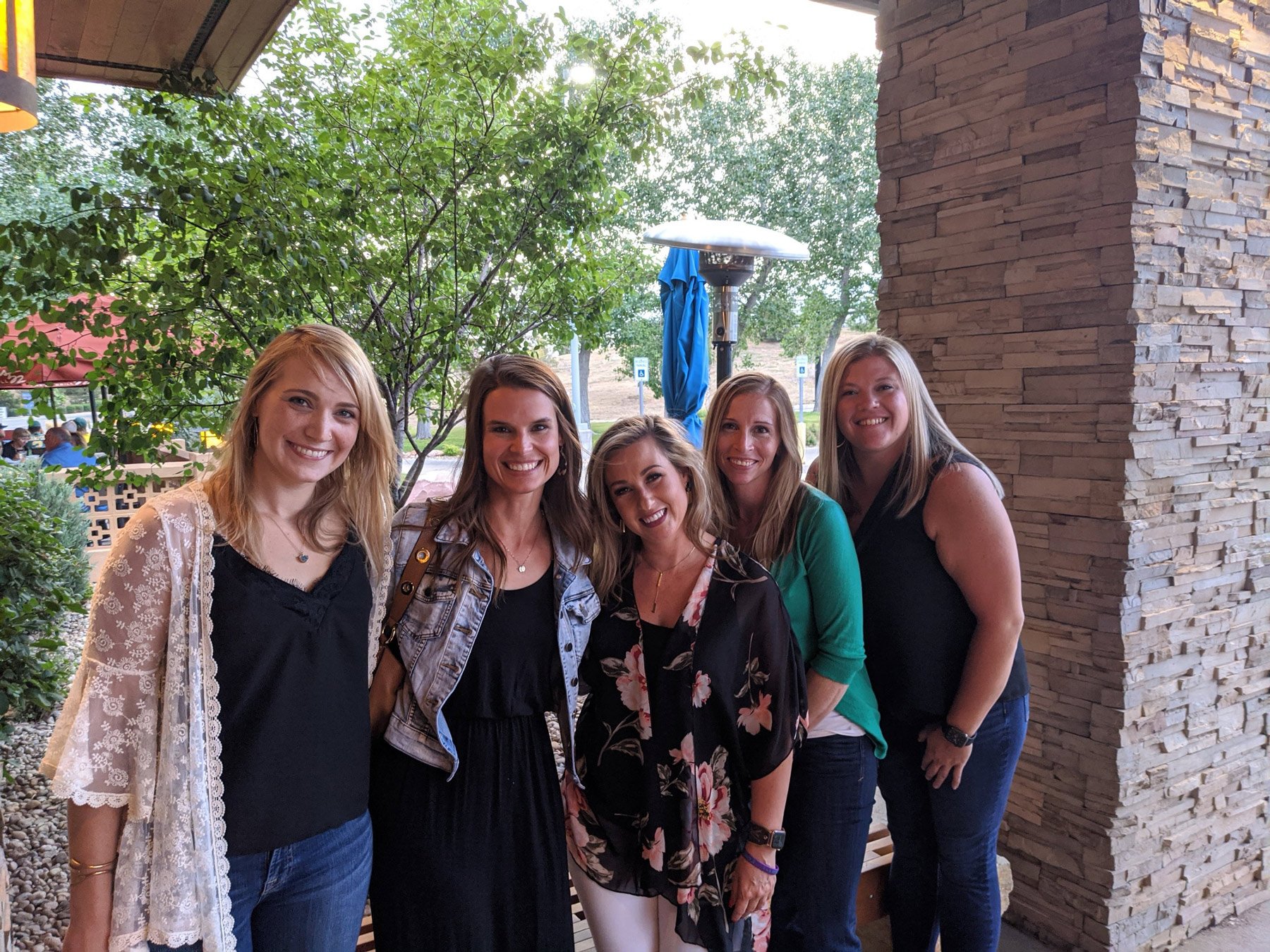In this photograph, five smiling women stand side by side outside, positioned in front of a stone column amidst a backdrop of trees, an umbrella, and a standing heat lamp. The women appear to be in their 30s or early 40s, all Caucasian, with a mix of blonde and brown hair. From left to right, the first woman has straight blonde hair, wearing a black shirt paired with jeans. The second woman sports straight brown hair and is dressed in a black dress with a jean jacket. Standing in the middle, the third woman has blonde hair and is wearing a black top adorned with pink flowers and white pants. The fourth woman, also blonde, is dressed in a green shirt and jeans. The fifth woman, a bit taller and physically more substantial, has blonde hair and wears a black short-sleeve shirt with jeans. They are all well-groomed, suggesting they might be dressed for an outing, and they pose with open, joyful smiles. The upper left-hand corner of the image reveals a bit of a wooden ceiling and a light fixture, hinting at an outdoor restaurant setting.